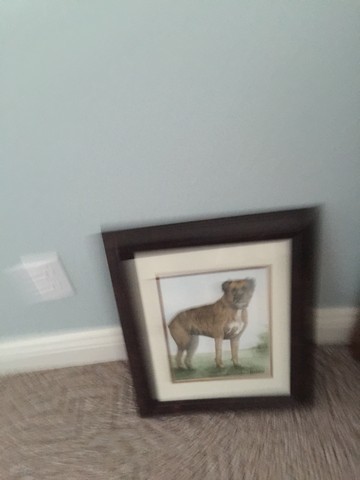The image showcases a wooden picture frame resting on a carpeted floor, adjacent to a blue painted wall. The frame, rectangular in shape with its length slightly exceeding its width, encloses a detailed drawing of a pit bull dog. The dog is depicted with a large black snout, brownish-black fur, a white chest, and a short tail, standing on a patch of grass. Surrounding the artwork is a white inner frame, which is further encased by the classic black wooden outer frame.